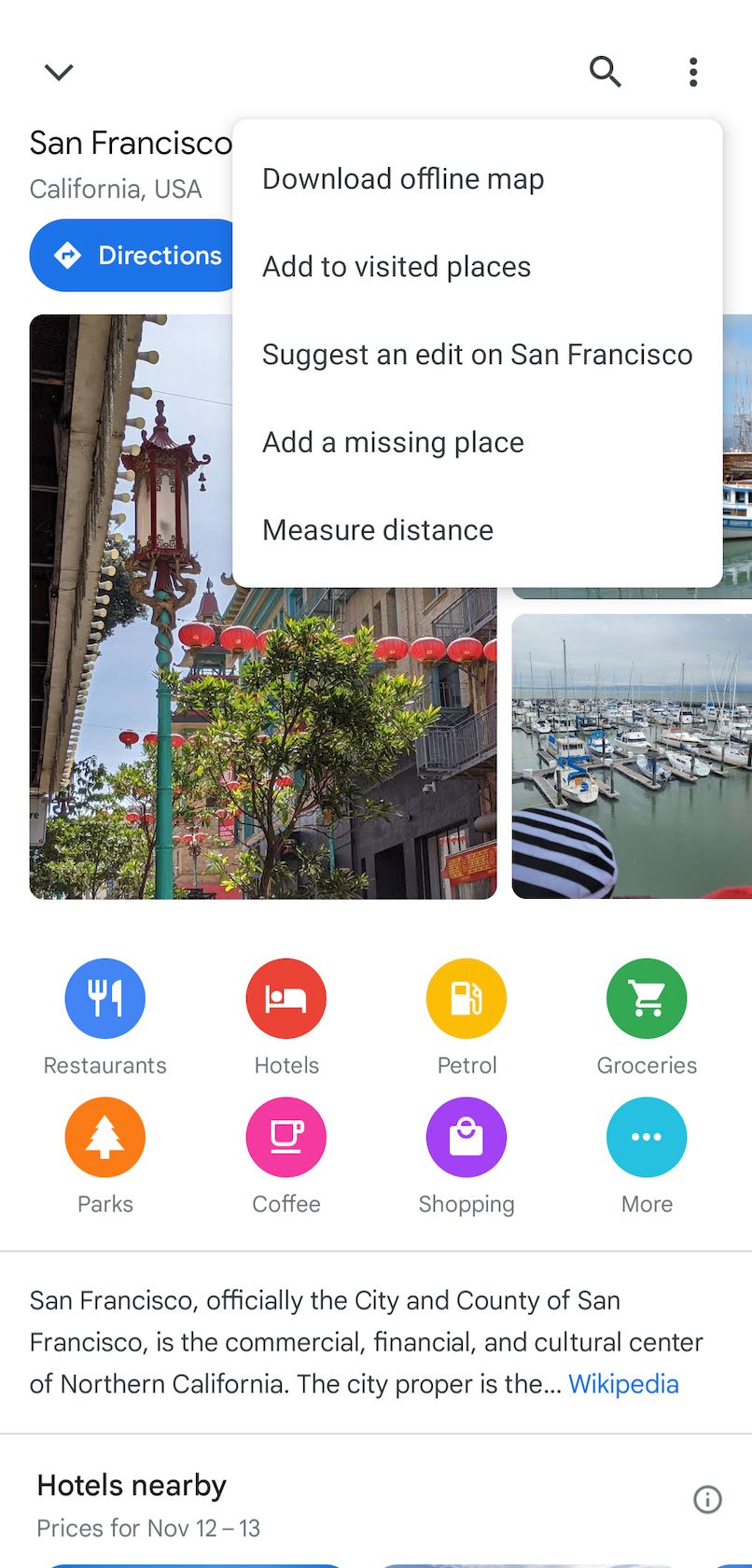The image is a detailed screenshot taken from a smartphone, focusing on a map interface displaying information about San Francisco, California, USA. At the top-left corner, a drop-down arrow is visible, while the top-right corner features a search bar and three vertically aligned dots. The label reads "San Francisco, California, USA," accompanied by a "Directions" button.

Below the three dots, an expanded drop-down menu provides options such as "Download Offline Map," "Add to Visited Places," "Suggest an Edit on San Francisco," "Add a Missing Place," and "Measure Distance." These menu options partially obscure three background photos, presumably showcasing scenes from San Francisco.

Beneath the photos, there are two rows of icons, each containing four icons. These represent various categories: restaurants, hotels, petrol stations, groceries, parks, coffee shops, shopping, and a "More" option.

A partially visible Wikipedia description starts with "San Francisco, officially the city and county of San Francisco, is the commercial, financial, and cultural center of Northern California. The city proper is the…" followed by an ellipsis, suggesting continuity, along with a clickable link to Wikipedia for more information.

At the bottom, there's a section highlighting nearby hotels with prices for the dates November 12th to 13th, though this section is cut off in the screenshot.